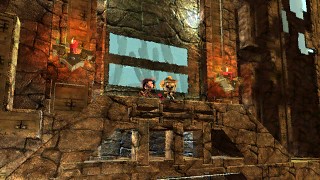The image depicts a video game scene featuring a slightly blurry skeleton-like character standing on a stone bridge. The bridge, which has four sections cut out beneath where the character is standing, spans the left and right sides of the image. On the wall behind the character, a torch emits a warm red-orange glow, casting a circular light around itself. Below this torch on the left side, there is a square wooden panel embedded in the wall, complete with a handle. Above the character, to the right, there is a stone carving resembling a turtle's head, hanging down from the wall. In the background, two large rectangular windows with blue panes reveal a view of towering cacti. Additionally, to the right of these windows, there are more windows with irregular shapes, also blue-hued.